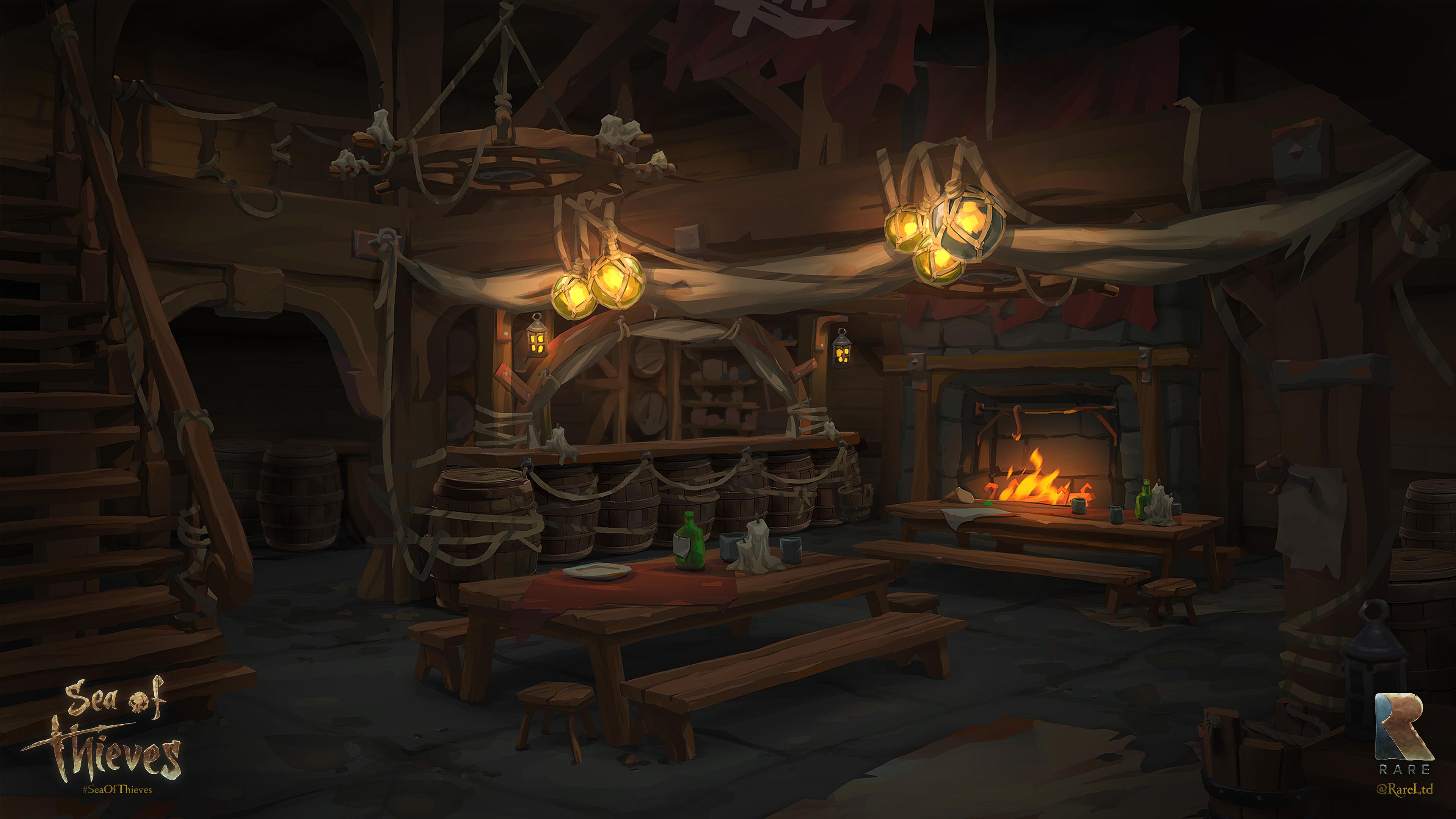The illustration depicts an interior scene from the video game "Sea of Thieves," set in what appears to be a fantasy or medieval-style tavern. The entire room boasts an intricate wooden design, including wooden walls, tables, stools, and a staircase on the left-hand side. Dominating the ceiling is a large wooden chandelier with two candle-lit fixtures hanging from it. The ambiance is dim, adding to the mysterious and cozy atmosphere.

In the center of the room stands a table draped with a red tablecloth, adorned with a white plate, green bottles, blue cups, and white candles. There is another table in the background, covered with a white tablecloth and similarly set with green bottles, blue cups, and white candles. To the right, a warm fireplace glows with orange and yellow flames, framed by a gray stone and wooden mantel.

The flooring consists of dark gray stone blocks. Overhead, a wheel is suspended by gray ropes, adding a nautical touch. Below, barrels line the bar area, alongside shelves holding various dishes. In the bottom left corner of the image, the text "Sea of Thieves" is displayed in stylized, gold letters. On the bottom right, a logo featuring a large "R" followed by "Rare LTD" in gold letters is prominently featured.